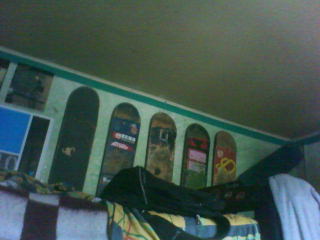The photograph captures a small bedroom from a low angle beside a bed, focusing on a wall with light green paint and a darker green stripe running along the top next to an off-white ceiling. Hanging vertically on the wall are five skateboards, each with unique designs and colors. The first skateboard is plain black, the second has a blue stripe with unreadable lettering, the third features a blue stripe without lettering, and the fourth presents a green background with multicolored stripes. The fifth skateboard displays a pink background with yellow and brown graphics. Additionally, there appears to be a couple of posters on the wall. In the foreground, a black backpack rests on a bed adorned with a white comforter patterned with burgundy crosses. A blanket or jacket is draped over the edge of the bed, contributing to the cozy yet eclectic room décor.